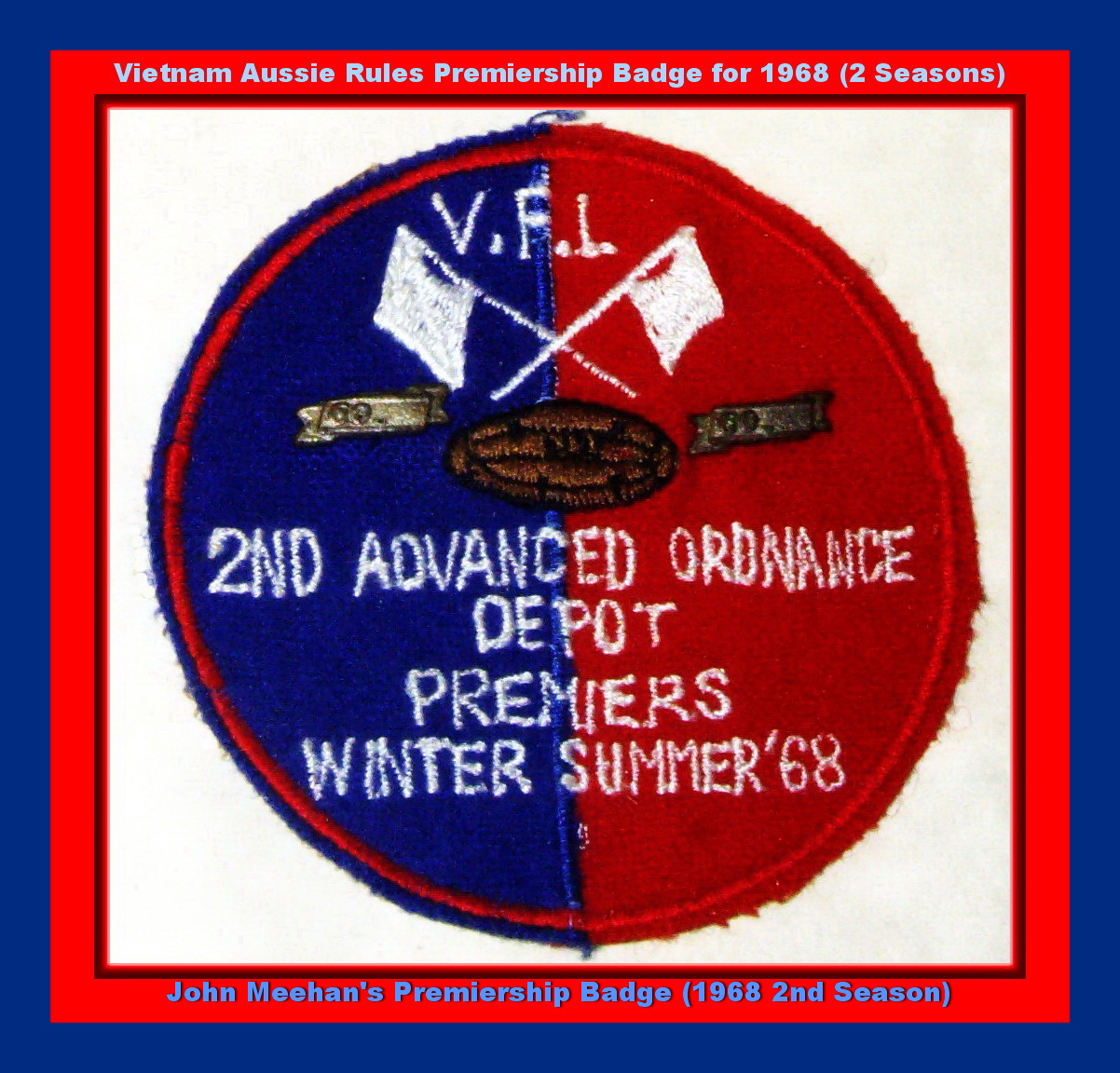The image showcases a patch that could be affixed to a shirt or jacket, prominently displayed in the center of the photograph. The patch is circular, with the left side in blue and the right side in red, featuring white text. At the top of the patch, it reads "VFL," with two white flags crossed beneath this text and a brown rugby ball just below the flags. The bottom half of the patch includes the text "Second Advance Ordnance Depot Premiers Winter Summer 1968."

Surrounding the patch is a white square, further framed by a bright red border with blue outer edges. The top section of the red border contains white text that says, "Vietnam Aussie Rules Premiership Badge for 1968, two seasons," indicating the context and history of the badge. The bottom section of the red border features blue text reading, "John Meehan's Premiership Badge, 1968, second season."

The badge itself is predominantly red, white, and blue, with a white background and central positioning in the image, representing the Vietnam Aussie Rules Premiership of 1968.